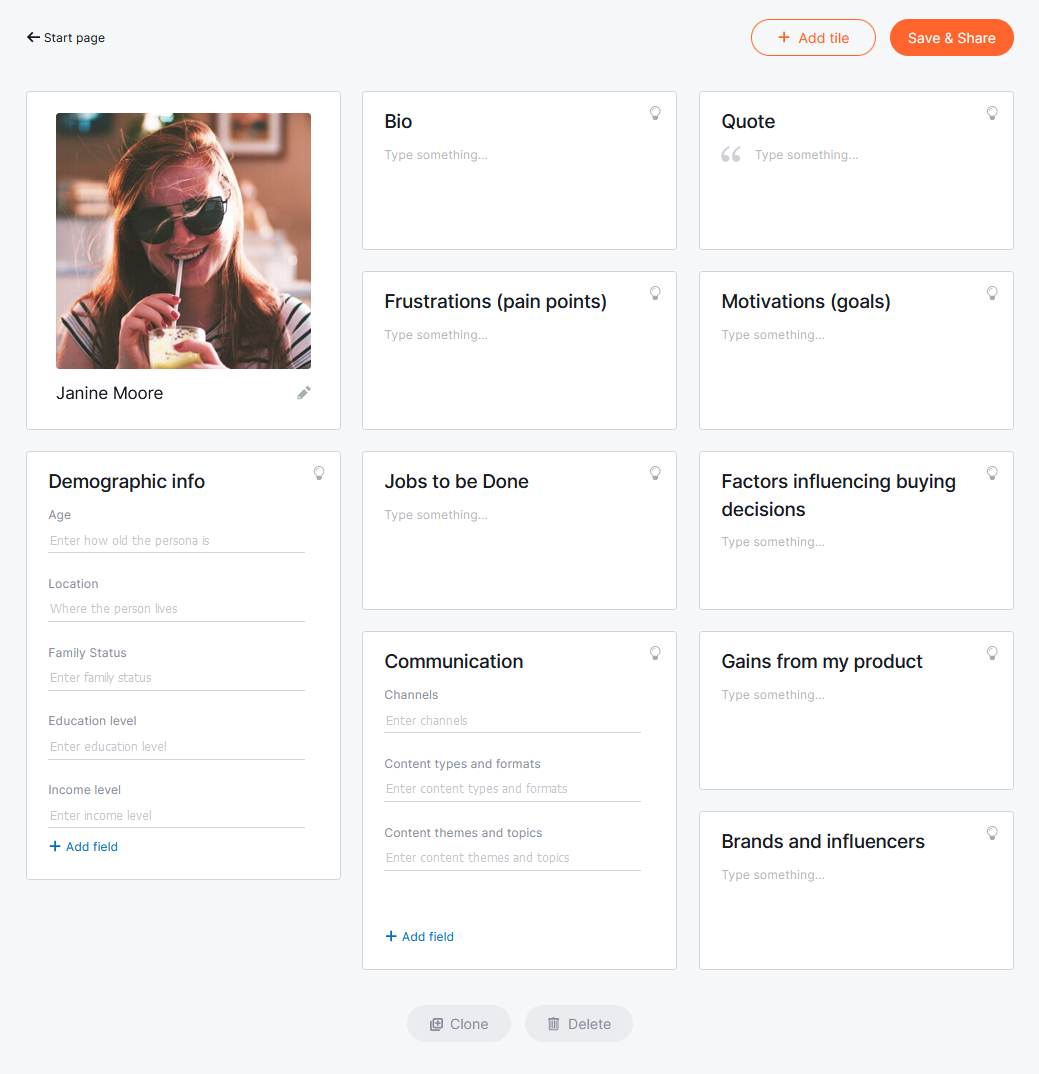The image captures a detailed view of a user interface on a web page, presumably a profile editing page. At the top of the page, there's a white banner with a "Start Page" label in black text and an accompanying black arrow pointing left. To the right of this banner is a white oval button with orange text, labeled "Add Tile" and featuring a plus symbol. Further to the right, an orange button is labeled "Save and Share."

Below this header, there is a prominent photograph of a woman named Janine Moore. She is smiling broadly, wearing black aviator sunglasses that partially conceal her eyes. Her vibrant red hair is swept elegantly over to the right, highlighting her cheerful demeanor. Janine is sipping from a straw held between her teeth, and her red-painted fingernails grasp a glass. She is dressed in a fashionable white and black striped shirt.

Next to her photograph, there is an empty bio section followed by a series of labeled sections— "Frustrations," "Pain Points," "Motivations," "Goals," "Jobs to Be Done," "Factors Influencing Buying Decisions," "Communication," "Gains for My Product," "Brand and Influencers"—all of which have not yet been filled in. 

Further down the page, demographic information fields are outlined for age, location, family status, educational level, income level, and ad preferences, though specific details are similarly unentered. At the bottom of the interface, there are functional buttons labeled "Clone" and "Delete."